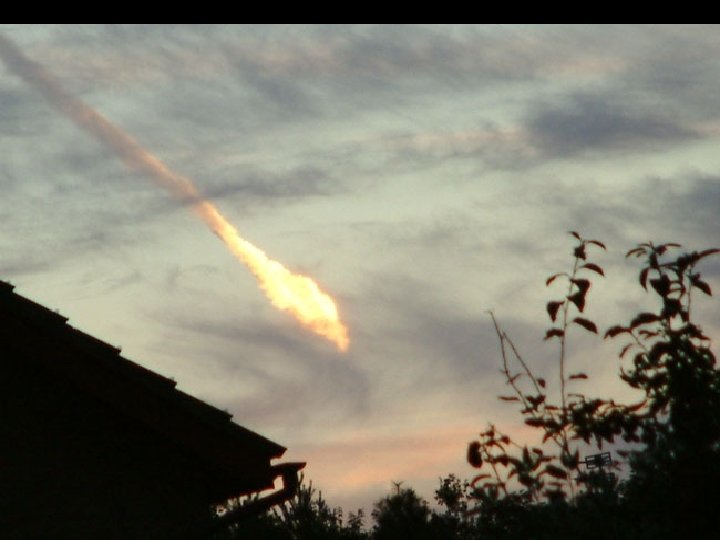This photograph captures a dramatic evening sky with a vivid display of colors and shadows. Dominated by dark, gray clouds that seem heavy but not rain-laden, the sky is tinged with hues of blue and, near the horizon, a touch of red and pink, signaling either a sunset or sunrise. Central to the image is a striking phenomenon: a bright fireball, emitting fiery yellow, orange, and white light, streaks through the sky from the top left corner to an oval-shaped intensification towards the middle. This fireball leaves a trail of smoke and dust in its wake, enhancing the dynamic feel of the scene. The ground features are silhouetted against this dramatic sky. On the left, the distinct outline of a roof's shutters or gutters is visible, while on the right, a cluster of shadowy vegetation and tree tops rise into view. This combination of natural and man-made elements, enshrouded in shadows due to the low light, provides a stark contrast to the fiery explosion in the sky.